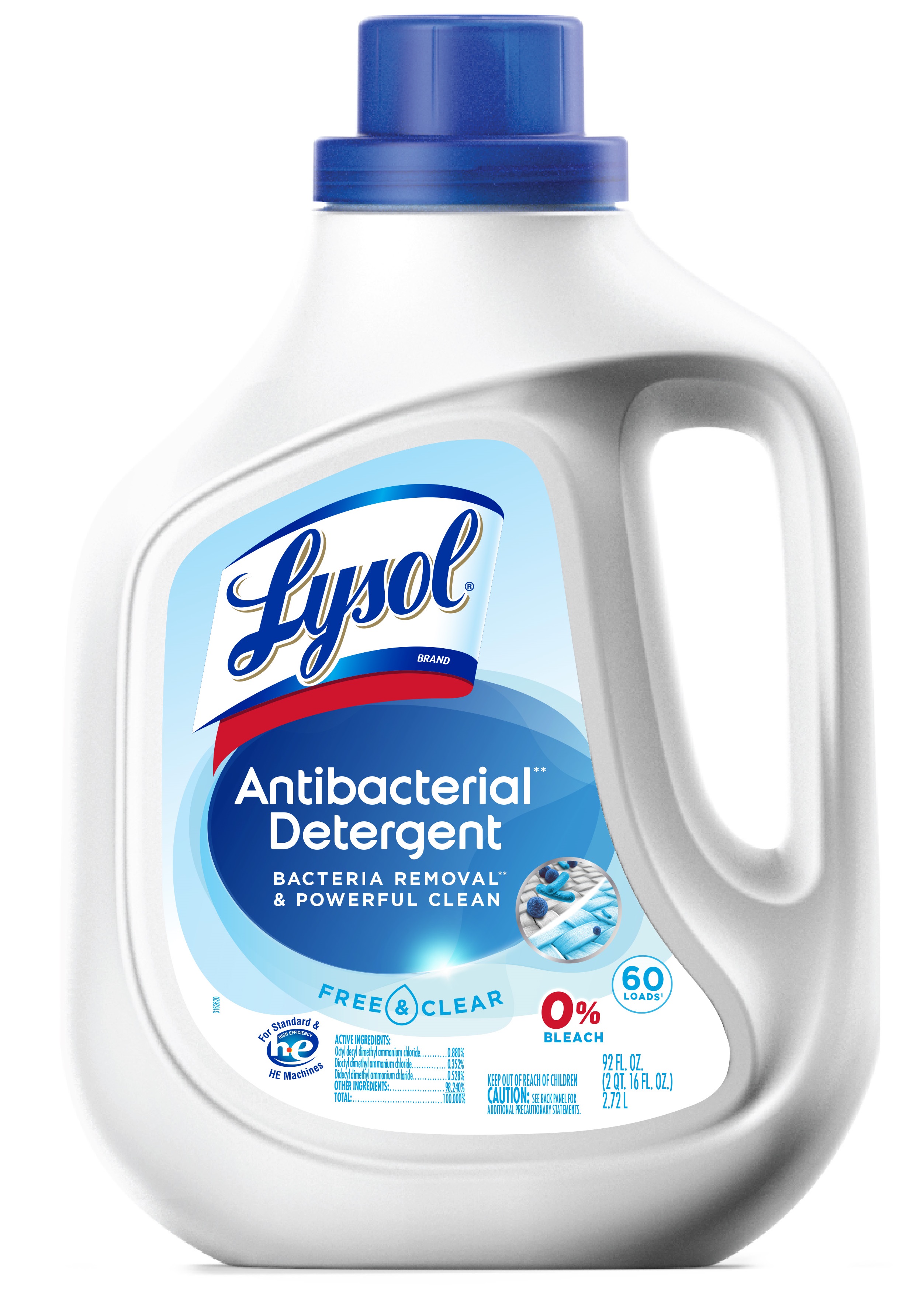This image is a highly professional product photo of a Lysol brand antibacterial detergent, set against a plain white background to highlight the product. The detergent is contained in a white plastic jug with a handle on the right side and a clear blue screw-on cap, revealing the spout underneath. The label is prominently displayed on the front, featuring the word "Lysol" in blue cursive writing on a white banner with blue edges and a red underline. Below that, the label details the product's features: "Antibacterial Detergent," "Bacteria Removal and Powerful Clean," and "Free and Clear." Additionally, it specifies "0% Bleach" in red lettering, indicating the product's bleach-free composition. A blue oval symbol on the label indicates that the detergent is sufficient for 60 loads. The label also mentions suitability for both standard and high-efficiency (HE) washers. The lower part of the label includes the product's ingredients and its volume, which is 92 fluid ounces. The overall presentation is pristine, with balanced lighting, contrast, and vibrant colors, typical of a retail-ready image suitable for platforms like Amazon or other online retailers.